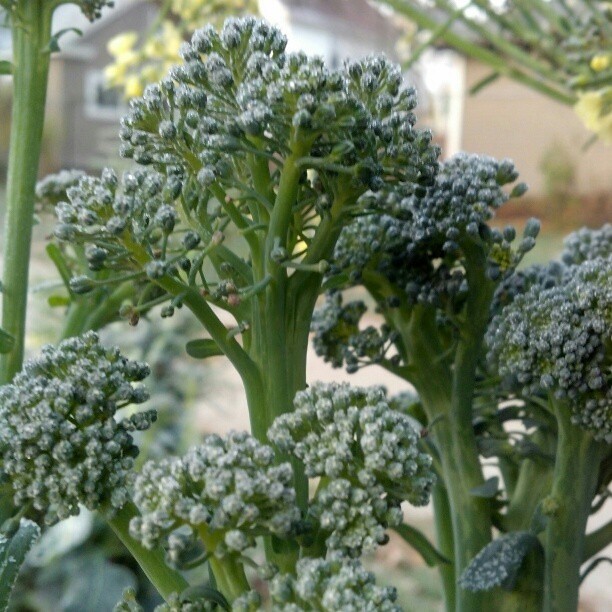In this outdoor daytime photograph, a collection of vibrant plants resembling broccoli dominates the foreground. The central focus is on several thick green stems that ascend from the ground, each crowned with cluster-like structures bearing a silvery-white hue, akin to frosty florets. These "broccoli-like" plants, with their characteristic branching stems, extend in various directions and are vividly detailed. In total, there are five prominent heads visible, each showcasing their unique arrangement of branches and buds.

The background, though blurred, reveals additional elements that add depth to the scene. A house can be seen, characterized by a grayish-brown wall and white-framed windows. Hints of another structure with a reddish wall and a slanted roof peek from behind it. Yellow flowers and green blades of grass add splashes of color to the periphery. This setting, suffused with natural light, highlights the rich green and silvery tones of the plants, making them stand out dramatically against the softly focused backdrop.